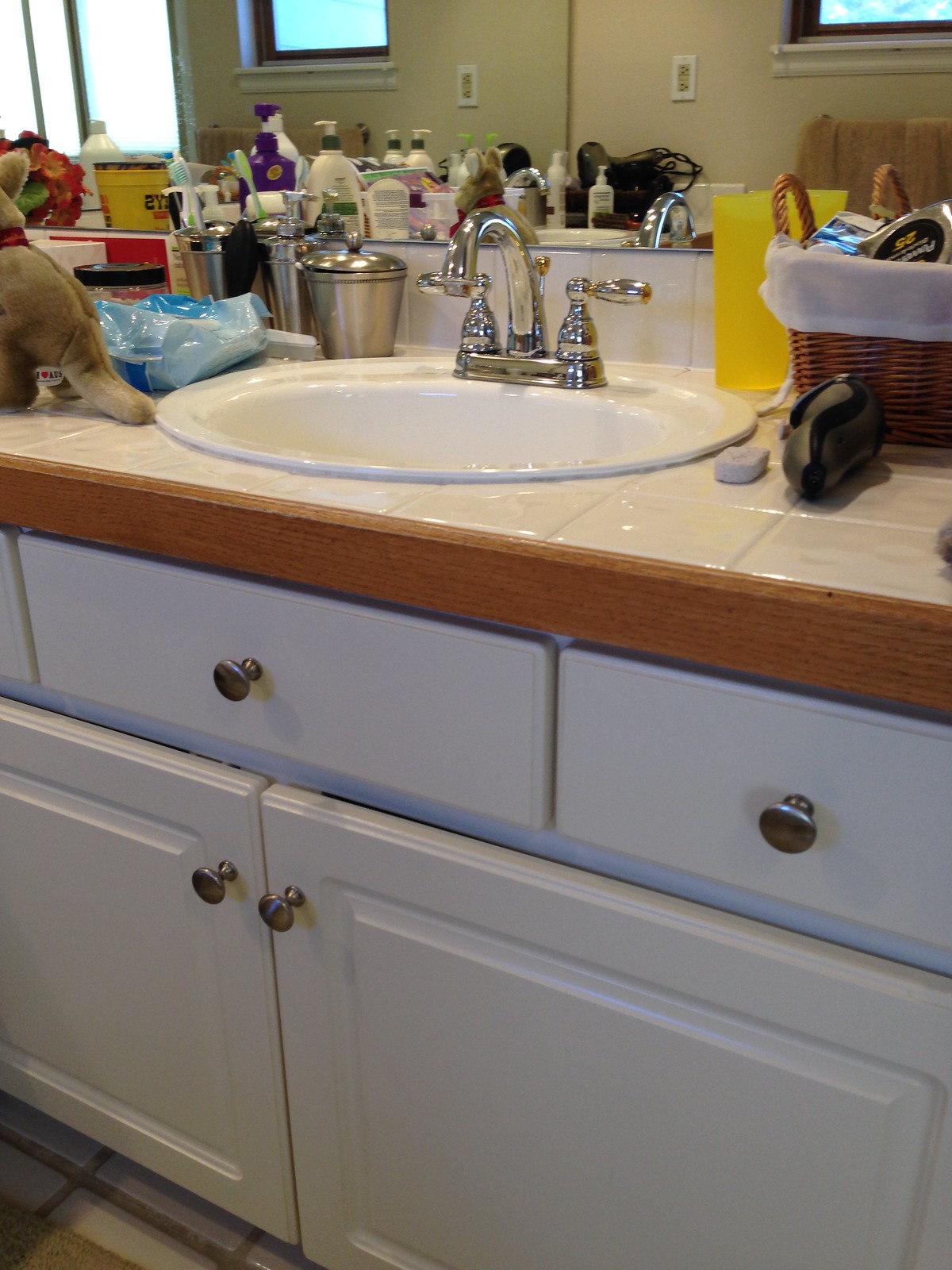This image showcases a white sink base with a golden faucet. The sink basin, also white, is complemented by steel handles. The countertop on the left side features a plush kangaroo toy, while the right side contains bins filled with shaving supplies. The backsplash is adorned with white tiles, and a mirror sits above the sink. Additionally, various sink accessories, including lotion and toothbrushes, are neatly arranged around the sink area.